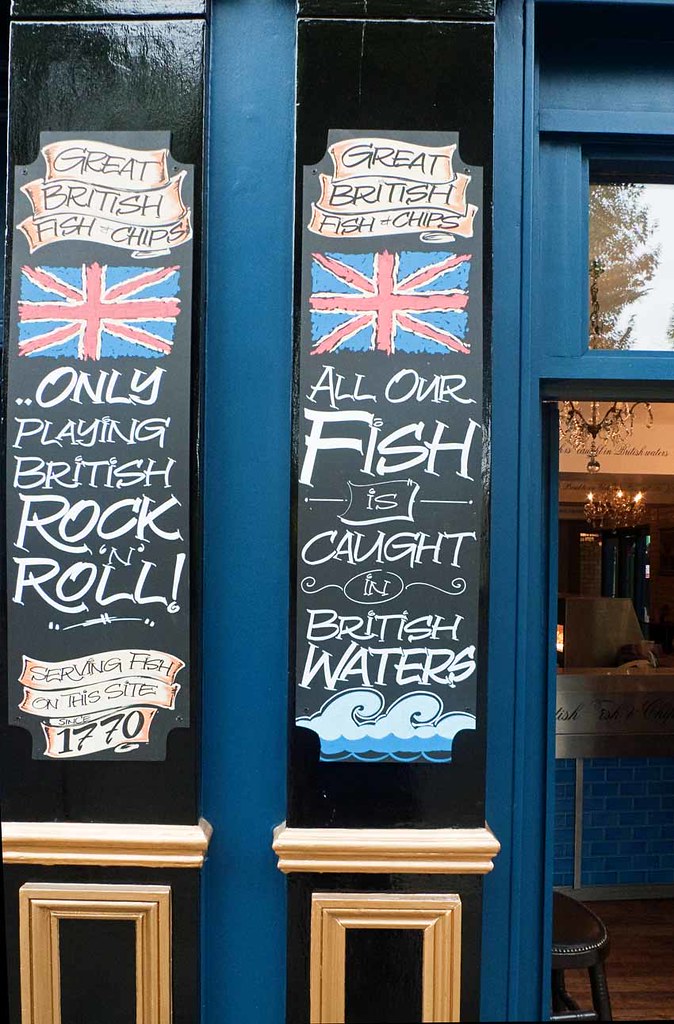The photograph captures the exterior of a traditional British pub, with distinctive vertical black panels resembling billboards rather than windows. The pub's entrance door, adorned in dark blue, is open, offering a glimpse of chandeliers hanging from the ceiling inside. The two prominent black panels flank the doorway. Each panel features a white-painted message in celebration of British culinary and cultural heritage. The left panel reads "Great British Fish and Chips" at the top, followed by a Union Jack and the phrase "Only playing British rock and roll." Further down, it states, "Serving fish on this site since 1770." The right panel mirrors the left with "Great British Fish and Chips" and a Union Jack, beneath which it declares, "All our fish is caught in British waters." The signage is detailed with wood-colored trim, contributing to the authentic, rustic charm of the pub’s façade.